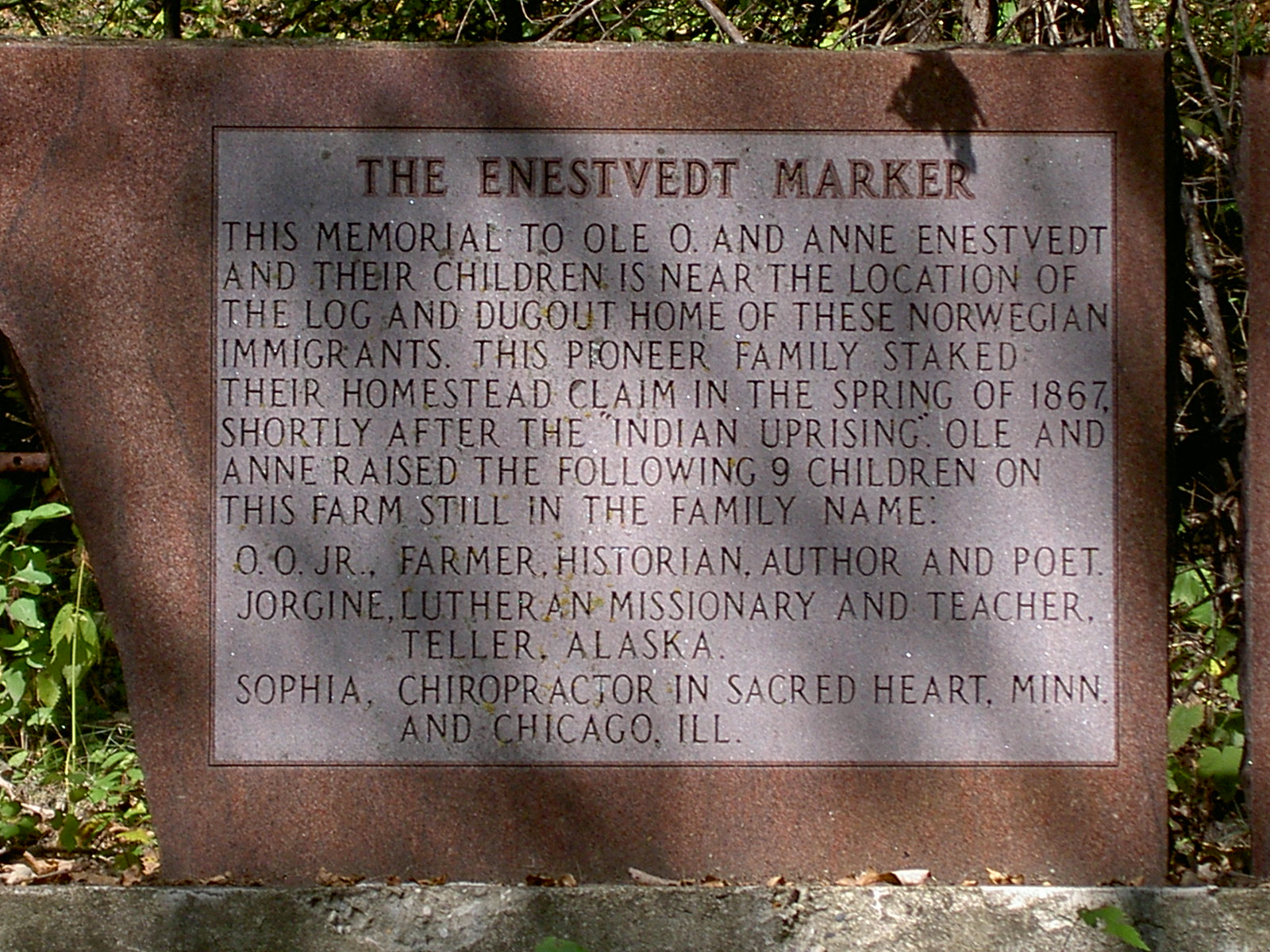This image features a large, smooth, brown stone monument set in a green and brown grass and dirt area with visible leaves, branches, and thin trees in the background. The monument, which appears to be sitting on another stone or concrete slab, is a wide rectangular shape with curved edges extending out of the frame. In the center of the stone is a pale gray rectangular engraving with reddish brown and black text. Across the top, it reads "Anestved marker." The inscription below in black lettering commemorates Ole O. and Anne Anestved and their children. It states: "This memorial to Ole O. and Anne Anestved and their children is near the location of the log and dugout home of these Norwegian immigrants. This pioneer family staked their homestead claim in the spring of 1867, shortly after the Indian Uprising. Ole and Anne raised the following nine children on this farm, still in the family name: Ole Jr., farmer, historian, author, and poet; Jorgen Luther, a missionary and teacher in Teller, Alaska; Sophia, chiropractor in Sacred Heart, Minnesota and Chicago, Illinois." The monument commemorates the significant history and legacy of the Anestved family.